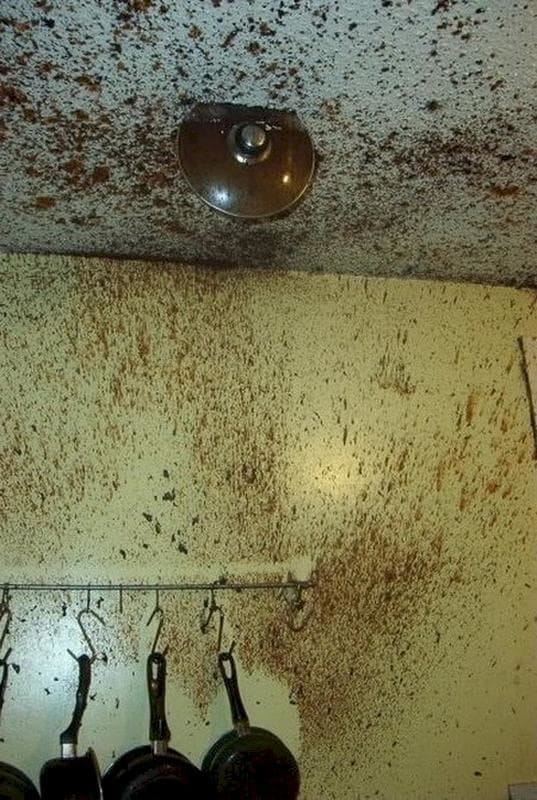The image captures a chaotic scene inside a kitchen, evident by the assortment of pots and pans hanging neatly from hooks on the wall—except for one missing pan, presumably the one in use. The focus of the photo is a culinary disaster: food is splattered everywhere, covering the walls and ceiling of the kitchen. The photo is taken from a low angle, emphasizing the unexpected trajectory of the pot's lid, which is lodged firmly into the ceiling, protruding by a fifth of its depth. The intensity with which the lid shot upward and became embedded in the ceiling suggests a significant pressure build-up in the pot. The splattered food forms a messy tableau, indicating that the contents of the pot were violently expelled. This perplexing and chaotic aftermath hints at a cooking mishap of considerable force, creating a daunting clean-up task.